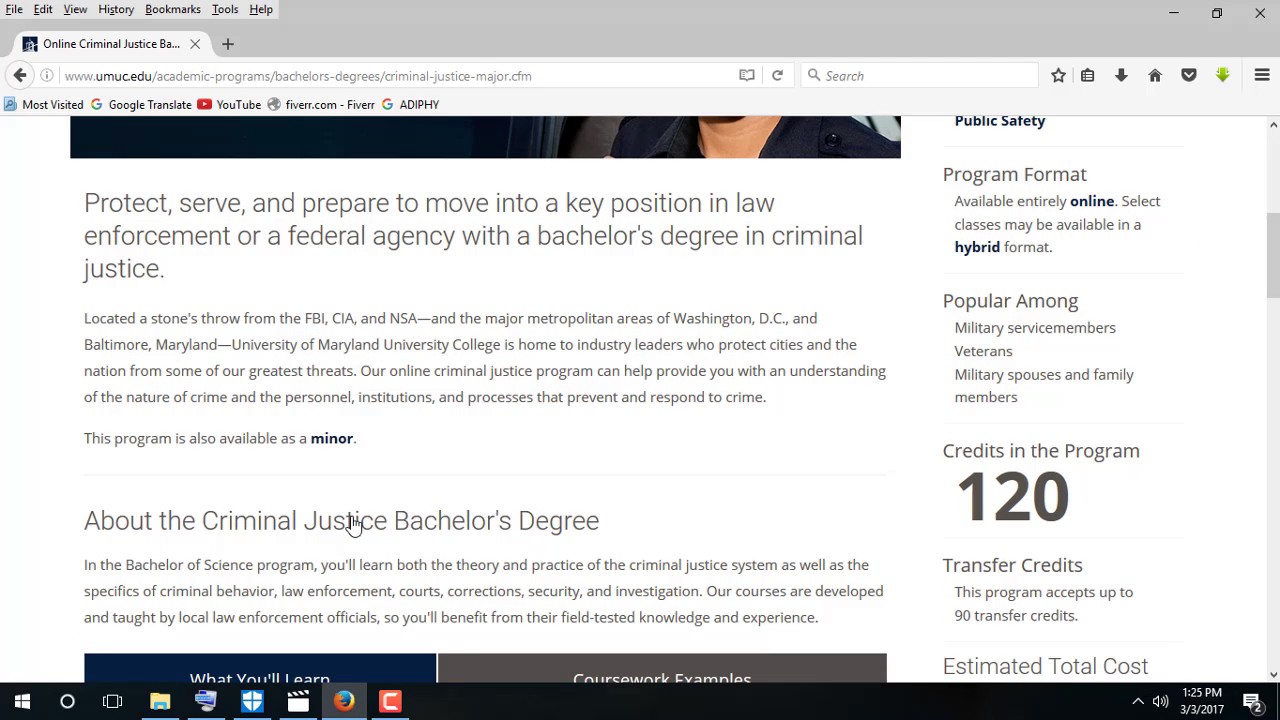**Detailed Caption:**

The screenshot captures a monitor displaying an educational website affiliated with the URL www.umuc.edu. In the browser tab, located at the top-left corner, there's a gray icon next to the text "Online Criminal Justice BA." The menu bar above the URL, featuring a gray banner, includes standard browser options such as File, Edit, View, History, Bookmark, Tools, and Help, all written in black.

To the right of the URL bar, there are several icons and features: a small white search window with a gray star for bookmarking, a checklist icon, a gray down arrow, a gray house, a gray pocket icon, an unfamiliar green icon, and three horizontally stacked black bars. Below this, there are commonly visited icons for Bookmarks, Most Visited, Google Translate, and YouTube. Additionally, the browser displays icons for Fiverr.com and a multicolored Google "G" logo that reads ADIPHY in bold black letters.

The main content of the webpage includes the heading "Protect, Serve, and Prepare to Move into a Key Possession in Law Enforcement or Federal Agency with a Bachelor's Degree in Criminal Justice." Following this, another heading reads "About the Criminal Justice Bachelor's Degree." On the right-hand side of the page, a sidebar titled "Public Safety" features sections for "Program Format," "Popular Among," and states that the program is 120 credits in bold black text. Below this, information about "Transfer Credits" and "Estimated Total Cost" is provided.

The bottom of the screen shows a taskbar typical of a Microsoft Windows operating system. The left side includes the Windows logo and icons for Phone, File Manager, a shield (likely Microsoft Defender), a movie clapboard, the Firefox browser icon, and an orange square with the letter "C." On the right-hand bottom corner, white icons show that the sound is on and display the time (1:25 PM) and date (March 3, 2017).